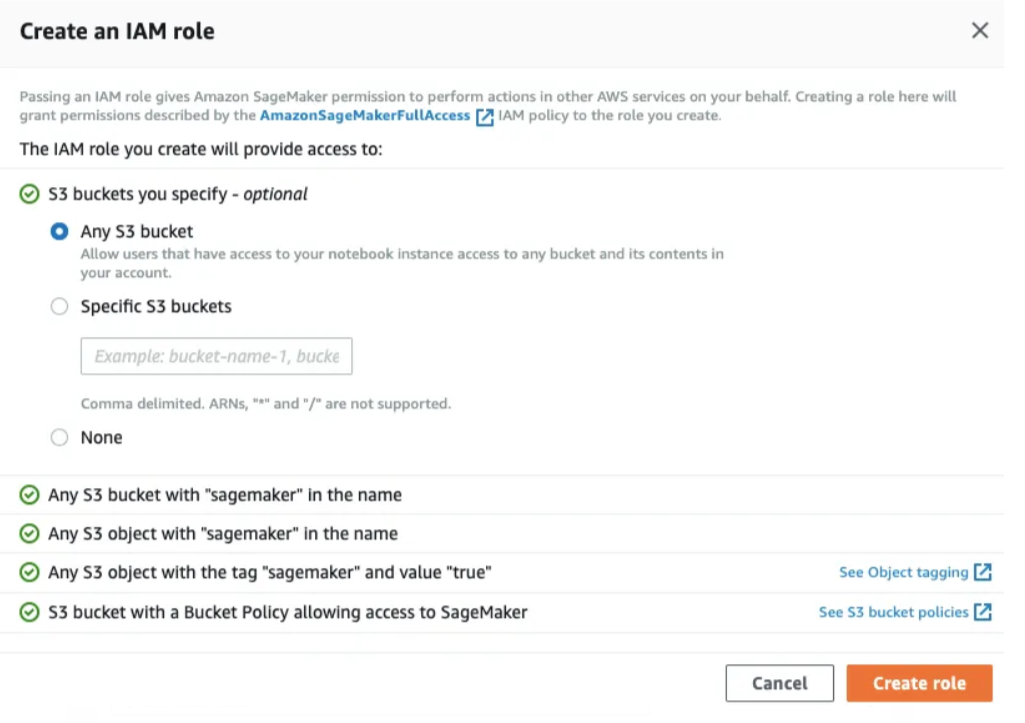Screenshot Caption: 

The screenshot displays the interface for creating an IAM role in Amazon Web Services (AWS), specifically for granting Amazon SageMaker permissions. At the top, it states, "Create an IAM role." Below, it explains that passing an IAM role allows Amazon SageMaker to perform actions on your behalf in other AWS services. It suggests creating a role that grants full access permissions to Amazon SageMaker. 

The interface provides options to specify S3 buckets, either allowing access to any S3 bucket with "SageMaker" in its name or any S3 object tagged with "SageMaker" and a value of "true." Additionally, users can specify a particular S3 bucket, for example, "bucket-name-1," to give SageMaker access to its contents. There is also an option to grant no S3 bucket permissions.

At the bottom, there is a button labeled "Create Role," which finalizes the creation of the IAM role with the specified permissions and settings. The screenshot appears to provide various customizable options for managing S3 bucket access and utilizing Amazon SageMaker services.